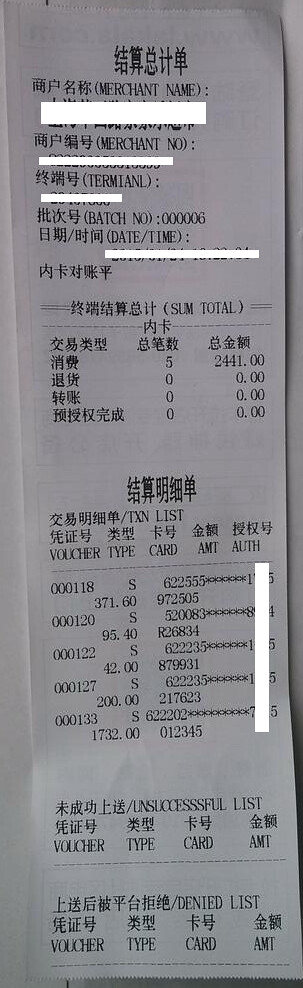This photograph captures a receipt printed on thermal paper, with several sections redacted using white boxes. The majority of the text on the receipt is composed of Asian characters. At the very top, a string of Asian characters is visible, likely indicating the name of the merchant or establishment. Below this text, another line of Asian characters followed by a parenthetical note (merchant name) is redacted. Further lines redacting the merchant number and terminal identification follow. The batch number, “00006,” is clearly visible. The date and time details are also obscured by a white box. 

In the middle section of the receipt, columns list various Asian characters interspersed with numbers, including “5” and “2441,” which may denote itemized charges or product identifiers. Toward the bottom of the receipt, the terms “list,” “voucher type,” “card amount,” and “authorization” are printed in English, indicating categorized transaction details. This image shows a detailed but partially redacted document, exemplifying both the specific transactional data typically found on a receipt and the selective concealment of sensitive information.